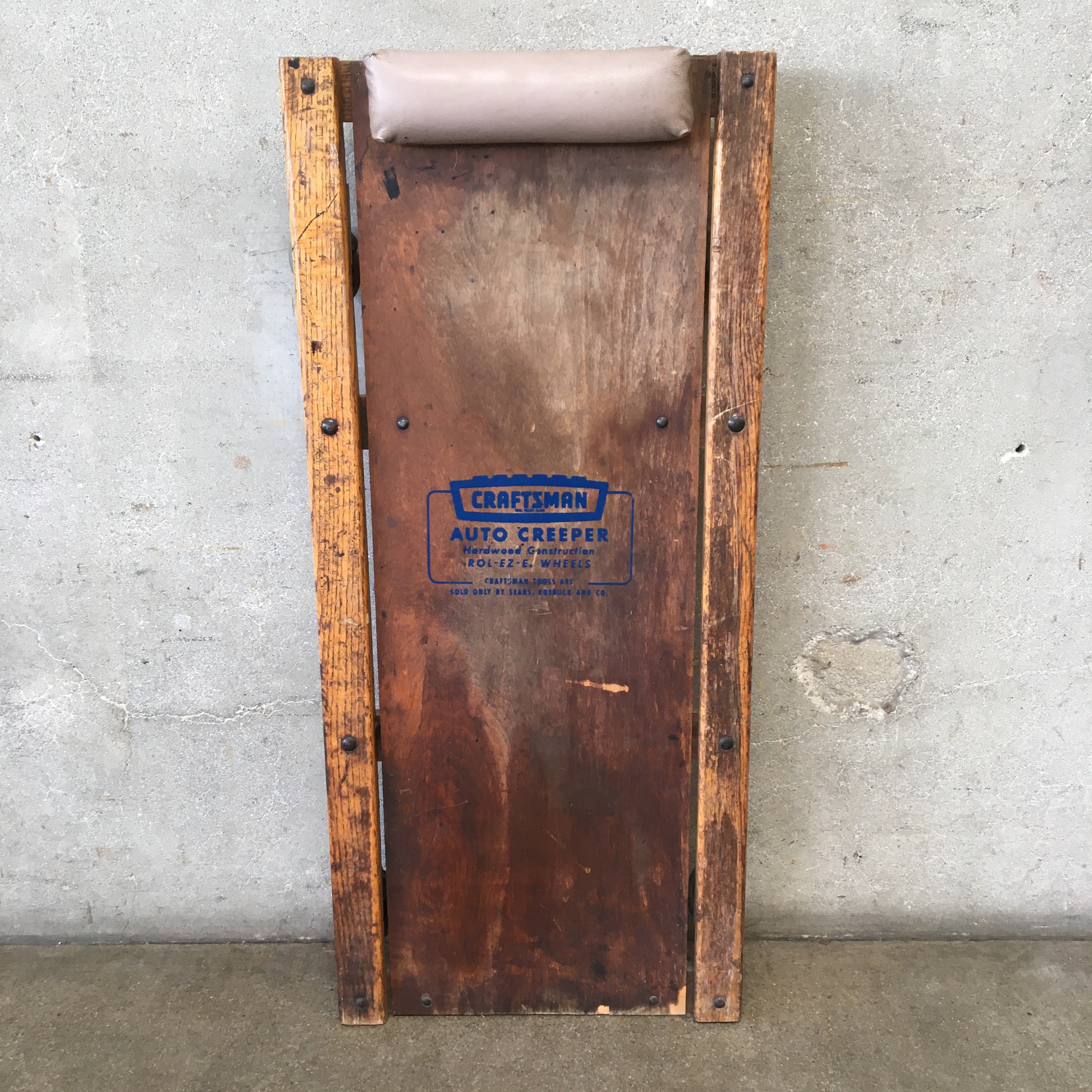This detailed photograph captures a weathered, dark brown wooden creeper, commonly used by auto mechanics to slide under vehicles. The creeper is entirely constructed from wood, except for a cushioned pillow at the top designed to support the head. The center of the creeper prominently displays the Craftsman logo and the label "Auto Creeper," along with descriptive text stamped in blue ink that reads, "Craftsman Auto Creeper, Hardwood Construction, Roll EZE Wheels." The creeper rests against a light gray colored wall, with a dark brownish beige colored ground in the foreground. The well-worn appearance of the creeper suggests it has seen extensive use and exposure to the elements.